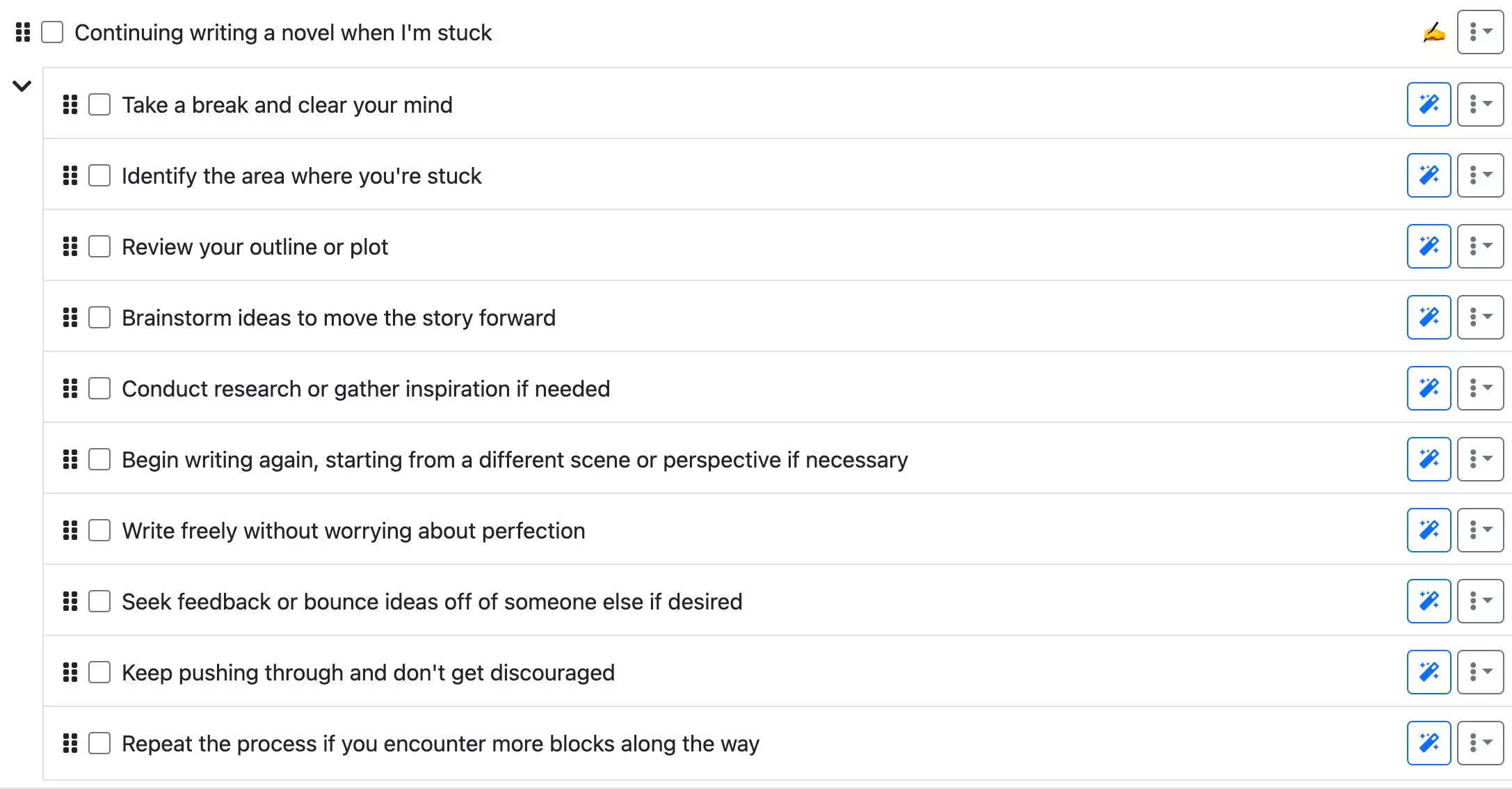The image depicts a user interface with various interactive icons and options. On the right-hand side of each row, there are two buttons: a vertical three-dot menu in gray and a drop-down menu represented by a gray square. These menus are positioned at the far right of each line.

To the left of the three-dot menu at the top row, there's an icon of a hand holding a pencil, symbolizing writing or editing capabilities. Adjacent to this, each row also features a blue sparkly magic wand icon, enclosed within a blue square, suggesting an additional functional tool or feature.

The left side of each row contains white checkboxes, all currently unchecked. Next to each checkbox, six black squares are stacked into two columns of three, likely signifying draggable elements or list organization icons.

The rows are labeled with motivational prompts and actionable steps for overcoming writer's block. The listed options are as follows:
1. "Continue writing a novel when I'm stuck."
2. "Take a break and clear your mind."
3. "Identify the area where you're stuck."
4. "Review your outline or plot."
5. "Brainstorm ideas to move the story forward."
6. "Conduct research and gather inspiration if needed."
7. "Begin writing again, starting from a different scene or perspective if necessary."
8. "Write freely without worrying about perfection."
9. "Seek feedback or bounce ideas off of someone else if desired."
10. "Keep pushing through and don't get discouraged."
11. "Keep the process if you encounter more blocks along the way."

This structured and icon-laden interface offers a comprehensive list of solutions and tools to aid writers in overcoming creative obstacles.